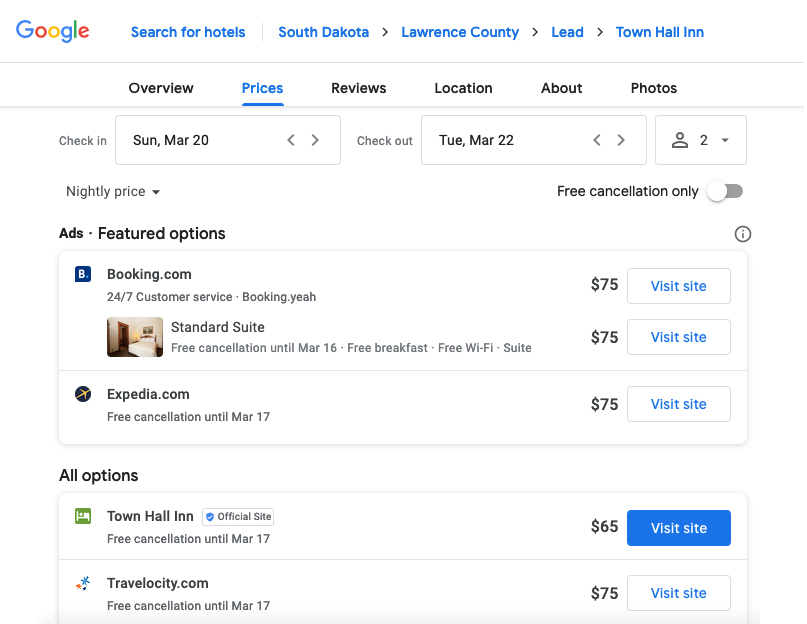The image depicts a detailed illustration of a Google search results page for hotels. The user has filtered options to a specific region, focusing on categories such as South Dakota, Lawrence County, and LEED. Featured prominently is the Town Hall Inn among the listings.

Subcategories at the top include tabs like Overview, Prices, Reviews, Location, About, and Photos. On the Prices tab, there are fields for inputting check-in and check-out dates as well as the number of adults staying. Once these details are provided, the page displays a variety of hotel pricing and listing options.

At the top, there's a section marked "Knightly Price," though it's unclear what this feature entails. The initial listings are sponsored ads, with "Featured Options" showing prices from Booking.com and Expedia.com, both offering a Standard Suite for $75. 

Additionally, there's a filter option to toggle 'free cancellation' on and off. Among the non-sponsored listings, Town Hall Inn is available for $65. The image shows the cursor hovering over, or about to click on, another listing for Travelocity priced at $75.